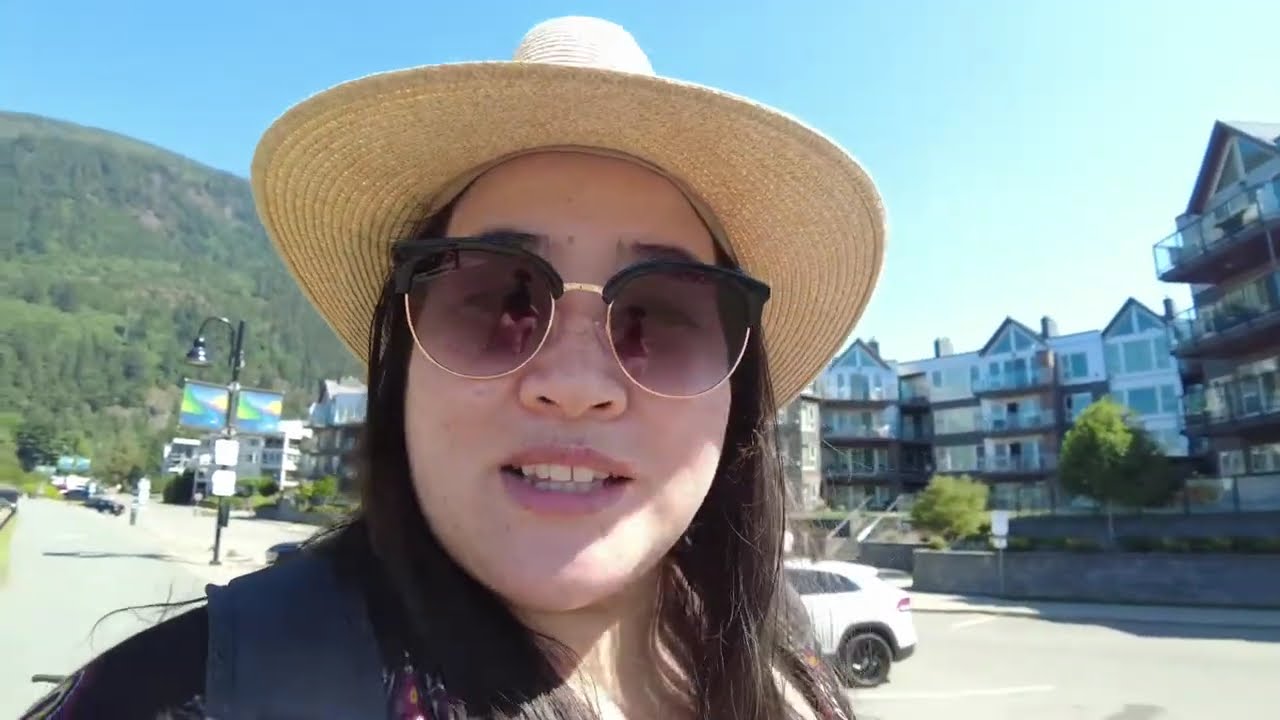In this bright and sunny photograph, the central focus is on a woman looking directly at the camera, with her face prominently featured in the middle of the image. She has long, dark brown hair cascading down her shoulders, and she’s wearing a beige straw hat with a circular brim. Her round, plump face is adorned with black-framed sunglasses that have a gold trim on the bottom, and she has pink lips with a glimpse of teeth, suggesting she’s mid-sentence or slightly smiling. She’s wearing a black blouse with some unknown pattern and has a backpack with a blue strap.

In the background, to the left, there's a large, raised hill covered in green trees. In front of the hill is a light gray street with no visible objects on it. On the right hand side, there are multi-story buildings that look like apartments or townhomes, primarily white with some light green or red brick accents. These buildings have extensive rows of windows, tall points at the top, and a large stone staircase leading up to them. A small patch of green grass, surrounded by concrete, is visible in front of the stairs. The upper right corner of the image features the front of a white passenger car. Additionally, you can see a bit of clear, light blue sky, adding to the brightness of the scene.